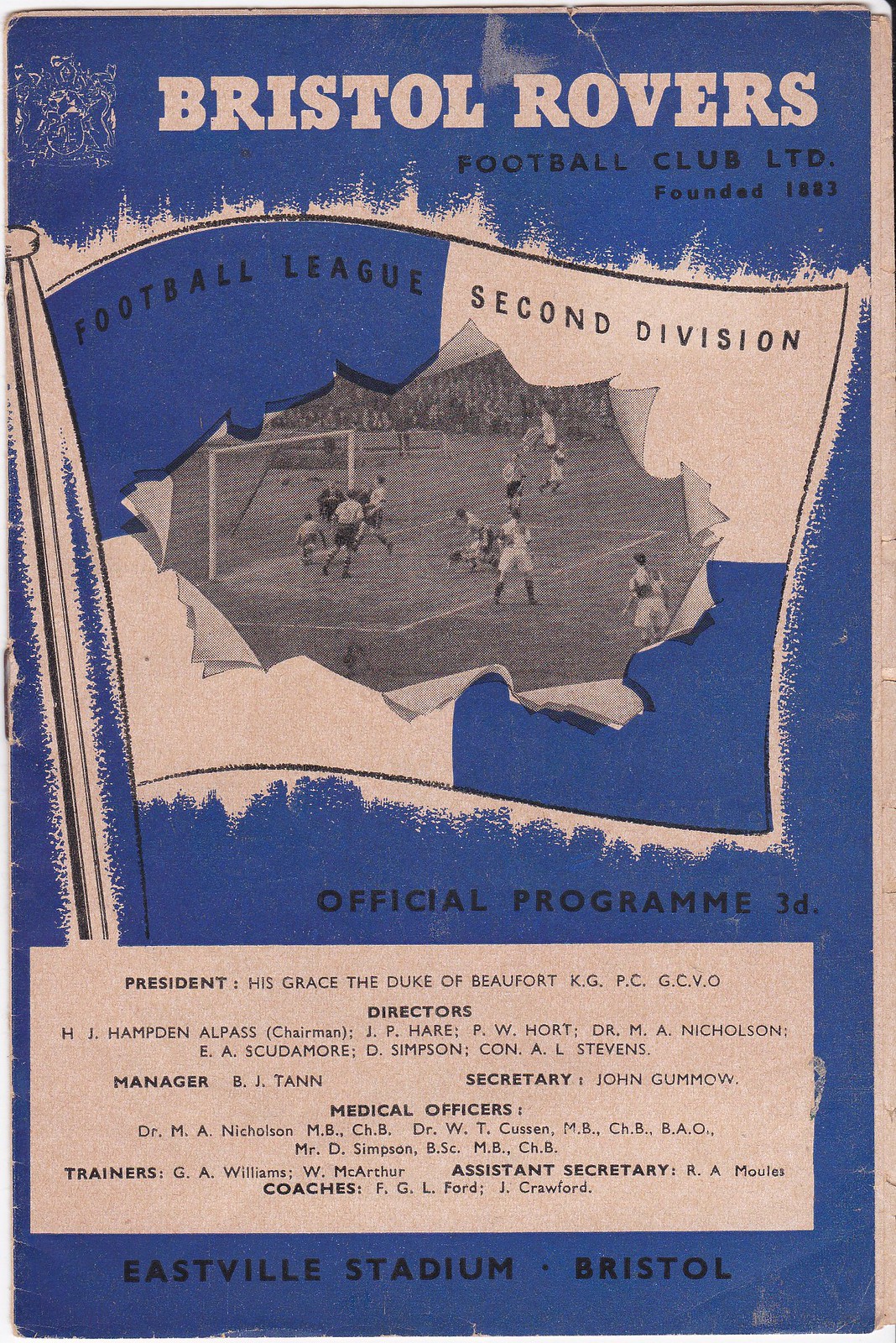The image is an aged flyer with a blue background and a worn paper-colored border, featuring the historic Bristol Rovers Football Club Limited, founded in 1883. At the top, it prominently states the club's name and founding year. Central to the design is a sketched flag divided into blue and white squares. Within the flag, there is a vignetting showing a live football game with several players and a goalie. "Football League" is written in the blue square, and "Second Division" is in the white square. Below this flag, it states "Official Program 3D." At the bottom, there's text indicating the venue, "Eastwell Stadium, Bristol," and a box listing club officials including the president, director, manager, secretary, medical officer, trainers, assistant secretary, and coaches. The flyer is slightly cropped, missing parts of the top and the right-hand side borders, but these details predominantly enrich its historical and nostalgic context.